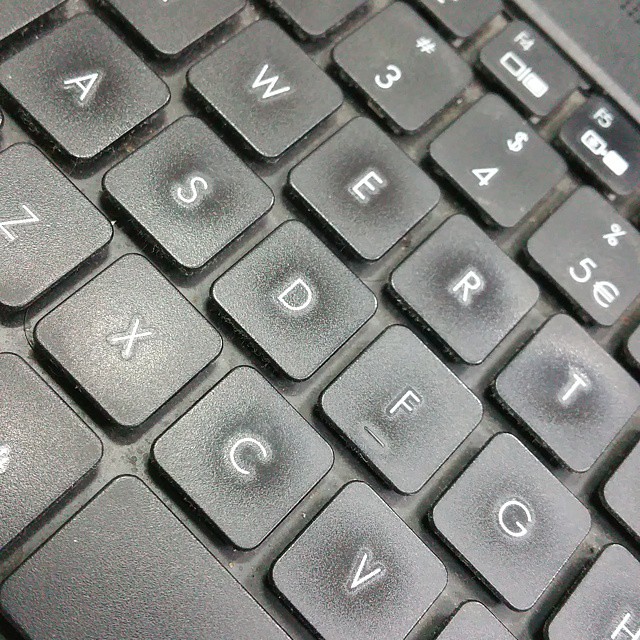This image is an extremely close-up, angled photograph of a worn and dusty black laptop keyboard. The visible keys are F4, F5, 3, 4, 5 (with a Euro symbol on the 5), W, E, R, T, A, S, D, F, G, Z, X, C, and V, along with a small portion of the space bar. The keys are black with white letters and numbers. The photo reveals significant wear and tear, particularly on the W, E, R, T, A, S, D, C, and V keys, with visible finger imprints and a greasy haze around them. Dust and debris are apparent between the keys, indicating the keyboard's age and need for cleaning. The image appears bright, likely due to a flash, and is taken at an angle, creating a diagonal, diamond-like composition. Blurred sections and a glimpse of the laptop's speaker holes at the top are also present.